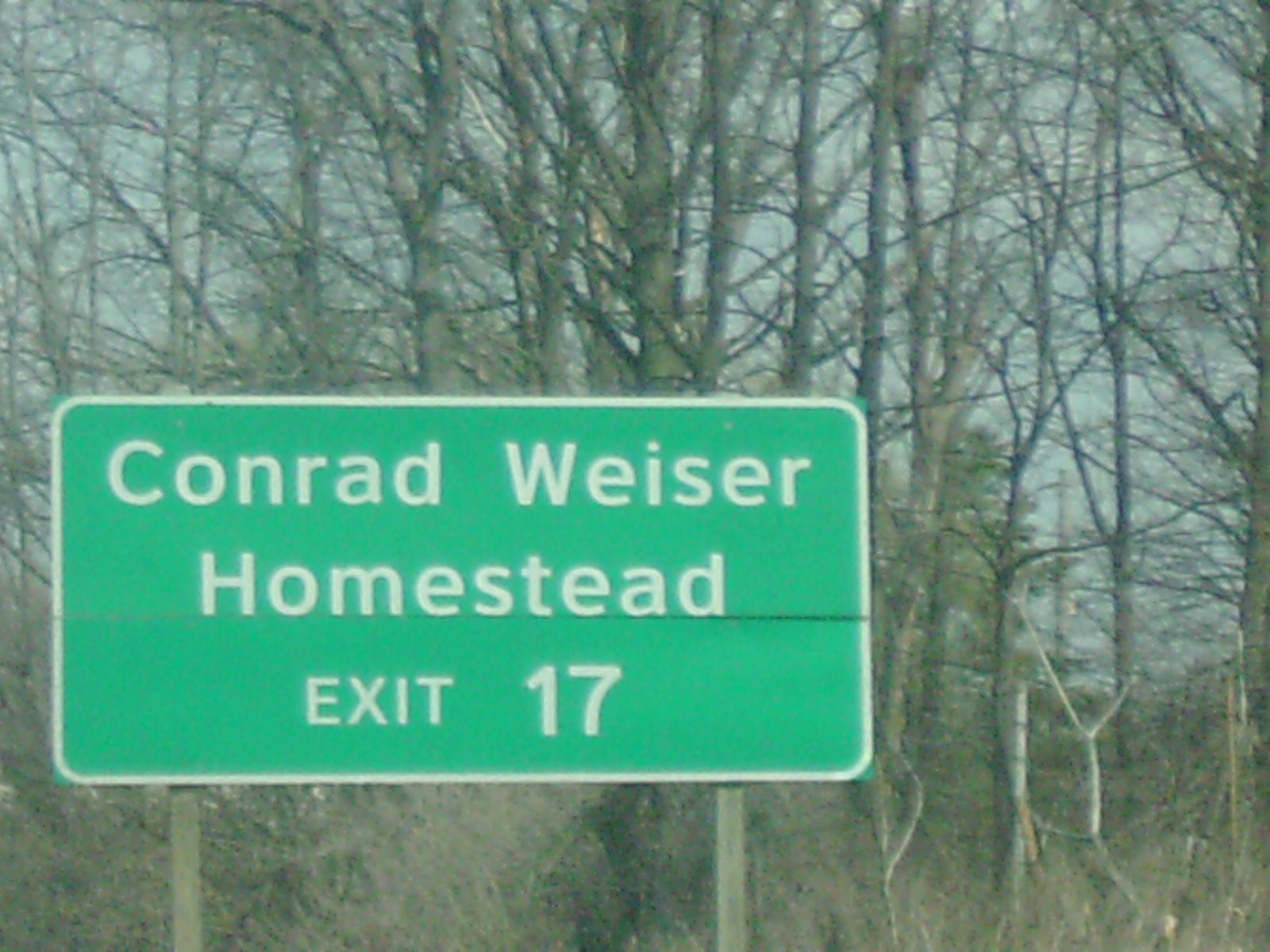This color photograph features a close-up view of a green road sign set against a barren, wintry background. The sign, an oblong shape typical of those found on U.S. interstates, state highways, and U.S. highways, reads "Conrad Weiser Homestead exit 17" in white letters. Surrounding the sign are numerous leafless trees, their bare branches intertwining and presenting a stark appearance suggestive of late fall or winter. The sky above peeks through the branches, its hazy and overcast nature implying a cool, sunless day. The proximity of the trees to the sign enhances the sense of desolation and quiet typical of a dormant season.